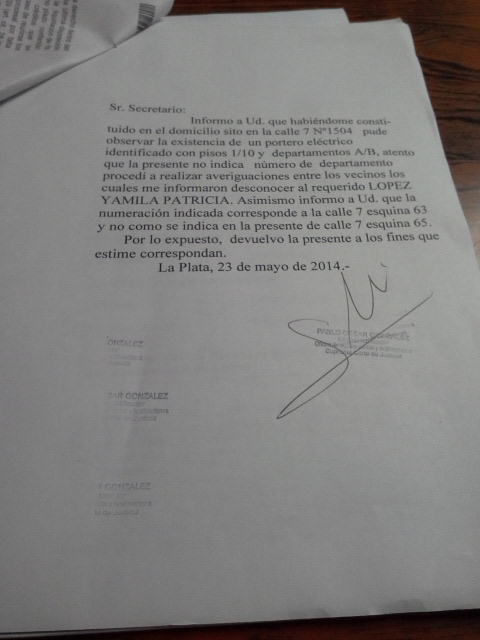This image depicts a white A4-sized paper with typewritten text in black ink. The paper is part of a multi-page document, evident from the top-left corner where it’s stapled and previous pages are folded over to reveal the current page. The document is written in Spanish and begins with “Senor Secretario.” The body of the letter includes paragraphs specifying details such as addresses and references to a portero eléctrico and various individuals. The closing line reads, “La plata 23 de mayo de 2014,” followed by a signature and stamps indicating official approval. The paper rests at an angle on a surface that appears to be a wooden table.